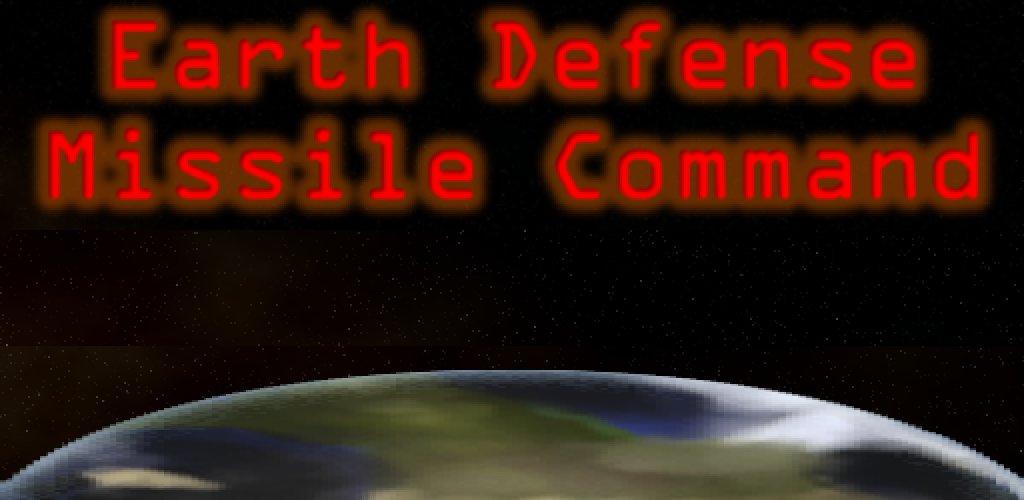The image appears to be a low-resolution, digitally generated screenshot from a video game or a 3D rendering designed to mimic a retro video game style, potentially dating back to the 90s. The lower portion of the image features a highly pixelated representation of Earth with various shades of blue, green, and tan illustrating the oceans and a fictional, non-realistic continent. This continent spans a wide area, resembling a landmass that could be interpreted as Asia or Eurasia, and it curves from the bottom left to the bottom right of the image. Above the Earth, the background is a stark black, dotted with small white specks representing distant stars in the space sky. The upper part of the image prominently displays red text with a faint red glow and brown border, spelling out "Earth Defense Missile Command" across two lines. The scene is enveloped in a nostalgic, early-computer-game aesthetic, characterized by its simplistic and pixelated graphics.